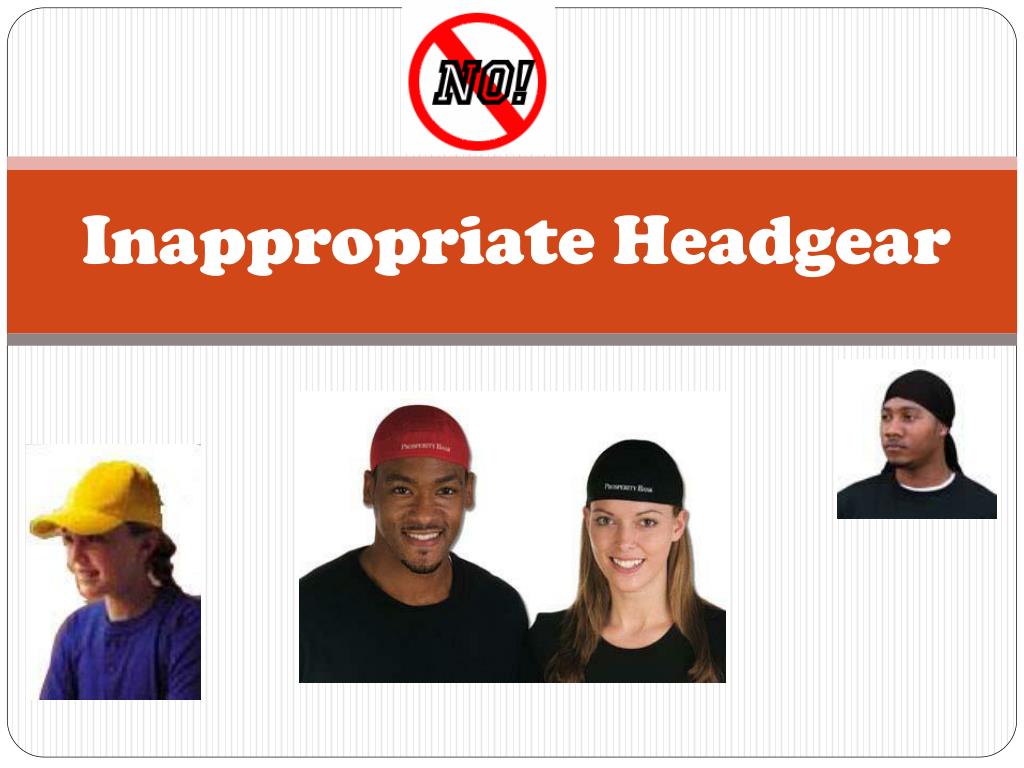The image is a detailed graphic design poster with a landscape orientation that combines color photography and typography set against a textured white and gray background with rounded corners, resembling a business or credit card. At the very top center of the image, there is a prominent red circle featuring a white interior and a diagonal slash going from the top left to the bottom right. Inside the circle, the word "NO!" is written in bold, black-outlined text.

Below this circle is a horizontal banner that spans the width of the image. The banner has a gradient background transitioning from lighter orange at the top to dark gray at the bottom. Centered within this banner are the words "inappropriate headgear" in bold white lettering.

Beneath the banner, there are three inset photographs of individuals displaying various types of headgear. On the left side, a young Caucasian girl with dark hair in a ponytail wears a yellow baseball cap and a cobalt blue sweatshirt, facing to the left. In the center, a young African-American man and a Caucasian woman stand side by side, both smiling brightly. The man, who has closely cropped hair and facial hair, wears a red headband with white text and a black rounded-neck T-shirt, while the woman with long light brown hair wears a similar black headband with white writing and a black rounded-neck T-shirt. To the far right, another young African-American man looks to the left, wearing a black do-rag and a black T-shirt with a white trim collar.

The overall artistic style of the image blends photographic realism with line art typography and illustration, effectively communicating the message about inappropriate headgear.